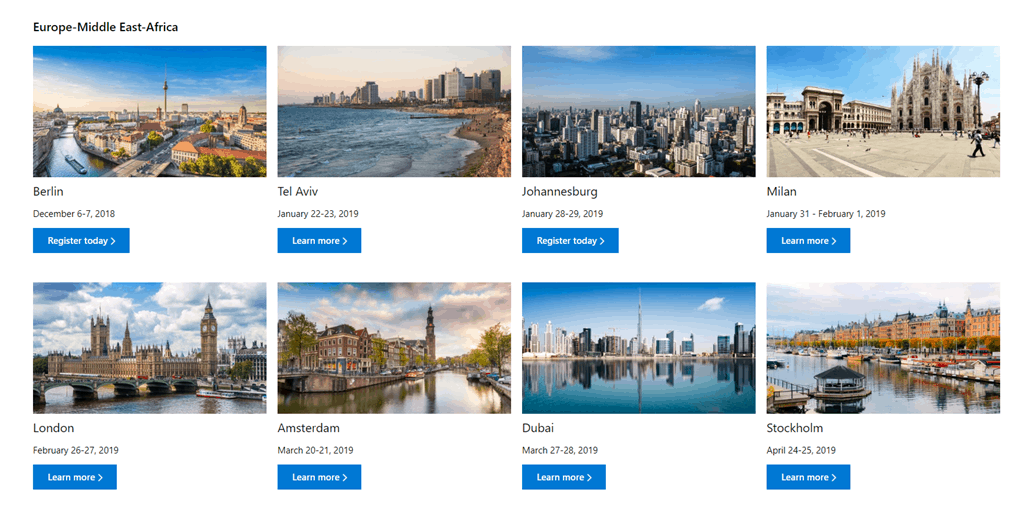The image is a screenshot taken from a desktop computer screen, showcasing a grid of eight individual images arranged in two rows, each containing four images. At the top left corner of the screenshot, the words "Europe, Middle East, Africa" are prominently displayed in black text.

Each of the eight images is accompanied by specific details below them. Underneath each image, the name of a city is written in black text, followed by a date, and then by a blue rectangular button that contains white text.

Starting from the top left, the first image in the first row has the city name "Berlin" written below it. Below "Berlin," the date "December 6, 2018" is listed. Beneath the date, there is a blue button with white text that reads "Register Today."

The second image in the first row...